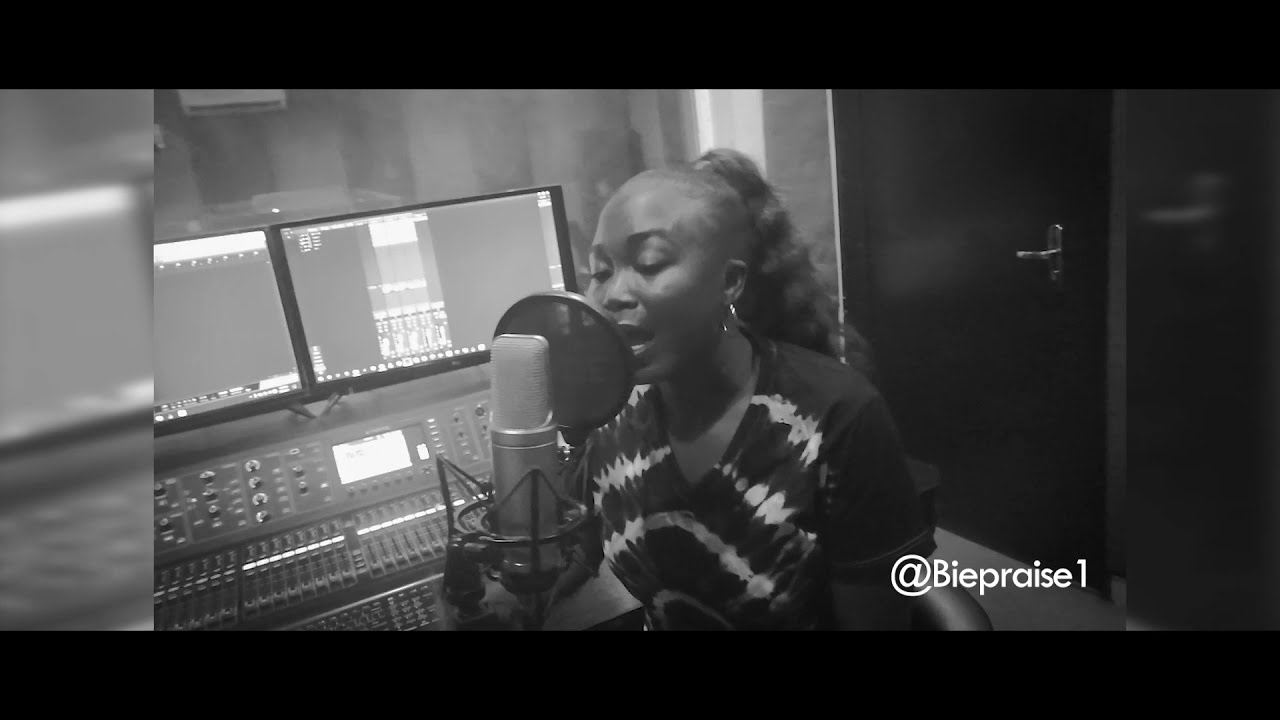This black-and-white image captures a young African-American woman in a recording studio, singing into a professional cylindrical studio microphone equipped with a windscreen. She stands at the center of the image, with her hair tied back and wearing earrings and a dark tie-dye t-shirt featuring a light-colored, horizontally curved pattern on the front. The background reveals a soundproof room with a black door featuring a silver handle, along with multiple computer monitors and a large mixing board, or audiovisual controller, filled with various buttons and dials. The studio setting is distinctly highlighted by these technical components. In the bottom right corner of the image, a watermark displays the username "@bpraise1."